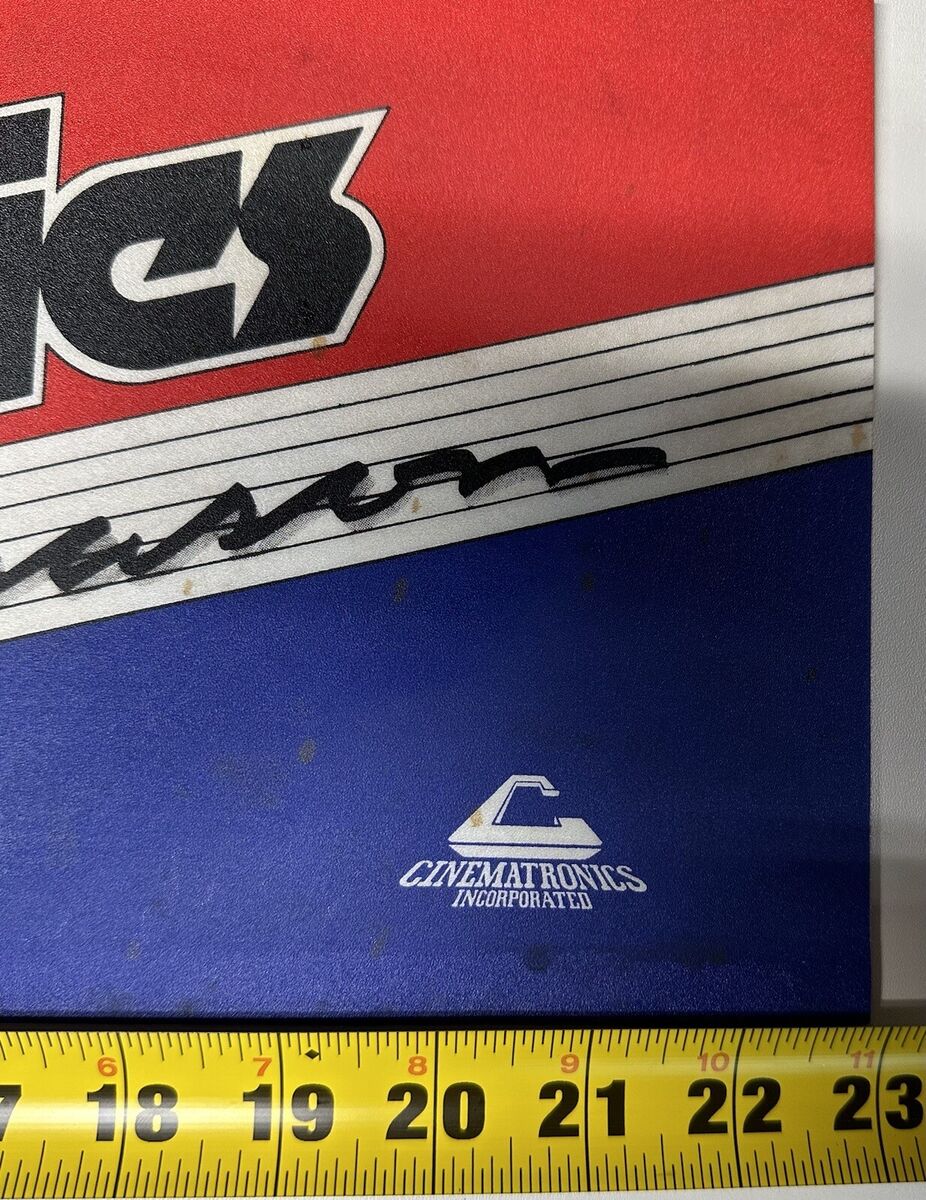The image depicts a partially visible sign or poster for Cinematronics Incorporated. At the bottom, a standard yellow tape measure stretches from 17 inches to 23 inches, indicating that the visible portion of the sign is approximately 6 inches across. Above the tape measure is a solid blue section featuring a large, angled letter "C" alongside the text "Cinematronics Incorporated" in white. Above the blue section, there's a white bar with an incomplete word written in black cursive, with some letters possibly reading "USON." This white section contains several black stripes. At the top of the image, a red diagonal section displays the black letters "ICS," which are bordered in white. The sign appears to be angled and is set against a white background, with a white border visible along the right edge of the image.